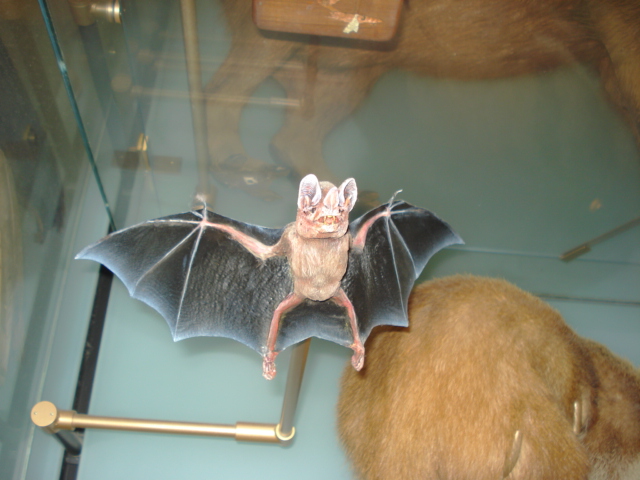In the image, taken through a clear glass display case, a real vampire bat is showcased with its wings fully outstretched. The bat is mounted on a stand resembling a copper pipe but painted in a metallic gold hue, giving it an industrial appearance. In the lower right corner, there is a mysterious furry object adorned with what look like gold tusks. Through the back of the glass case, the belly and back legs of a dog-like animal can be seen lying on the same surface, adding depth to the scene. The entirety of the display resembles a meticulously crafted diorama, featuring a bat and various other mammals, all contained within a series of glass cabinets.